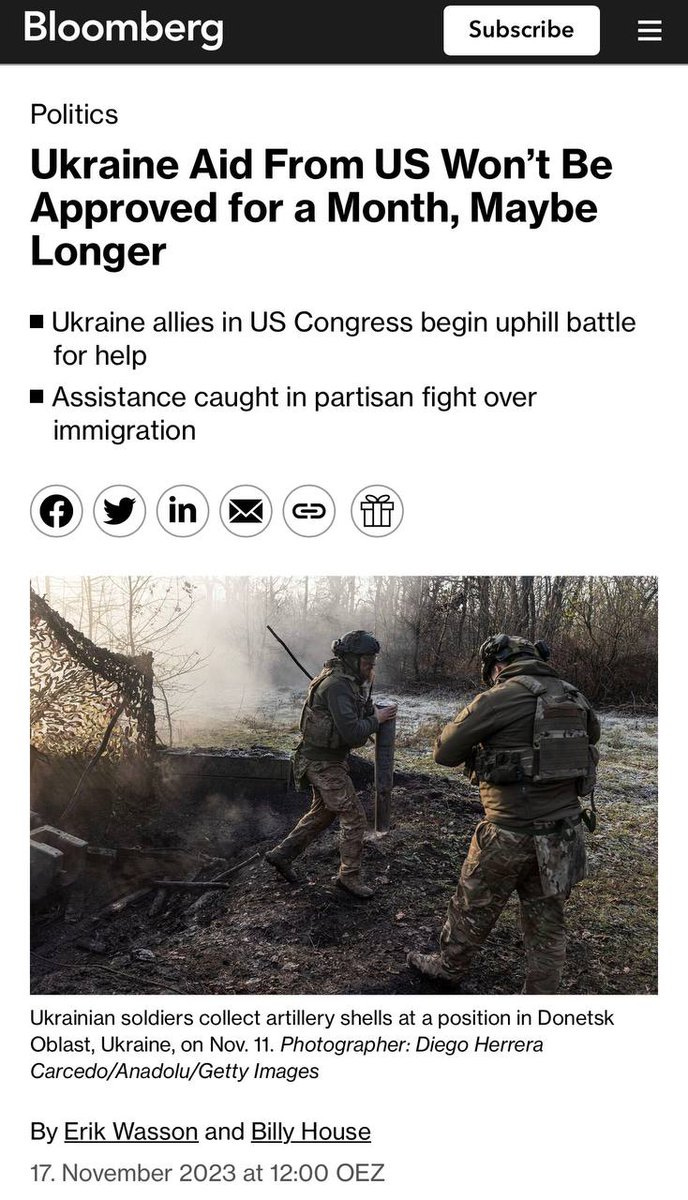At the top of the website, there is a black border with the word "Bloomberg" in white on the left-hand side. On the right-hand side of the black border, there is a white rectangle with the text "Subscribe" in black. Below this, the background transitions to white. In black text, it says "Politics."

The main headline reads:
"Ukraine aid from the U.S. won't be approved for a month, maybe longer."

Below the headline are two bullet points:
- "Ukraine allies in the U.S. Congress begin uphill battle for help."
- "Assistance caught in partisan fight over immigration."

Further down, there are icons in grey outlined circles for sharing the article, including Facebook, Twitter, LinkedIn, email, a general share symbol, and an unidentified gift/donate symbol.

The image accompanying the article shows two Ukrainian soldiers in a wooded area with smoke in the background. The caption beneath the image reads:
"Ukrainian soldiers collect artillery shells at a position in Donetsk Oblast, Ukraine, on Nov. 11. Photographer: Diego Herrera, Anadolu, Getty Images."

Additional text includes:
"By Eric Watson and Billy House."
"17 November 2003 at 12:00 OEZ."